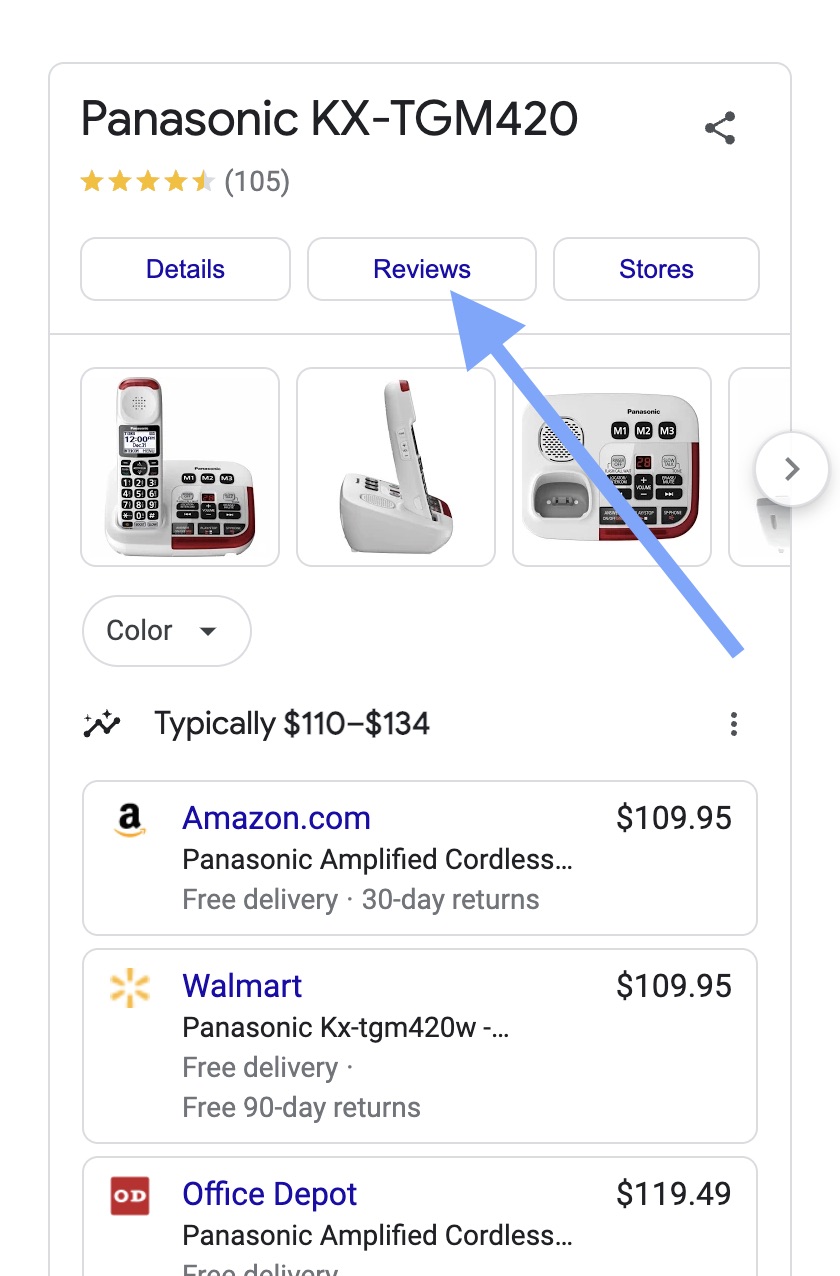The image features a white background and prominently displays a Panasonic KX-TGM420 phone, which is white with black and red trim. The phone has received an average rating of four and a half stars from 105 reviews. Beneath the phone, there are three rectangular sections labeled "Details," "Reviews," and "Stores," with a blue arrow pointing to the "Reviews" section.

Accompanying the image is a pricing and availability comparison from various retail stores:

- **Amazon.com**: 
  - Listed as the Panasonic Amplified Cordless.
  - Offers free delivery and 30-day returns.
  - Priced at $109.95.

- **Walmart**:
  - Listed as the Panasonic KX-TGM420W.
  - Offers free delivery and 90-day returns.
  - Priced at $109.95.

- **Office Depot**:
  - Listed as the Panasonic Amplified Cordless.
  - Offers free delivery.
  - Priced at $119.49.

Additionally, there are three vertical dots and an oval indicating a typical price range of $110 to $134.